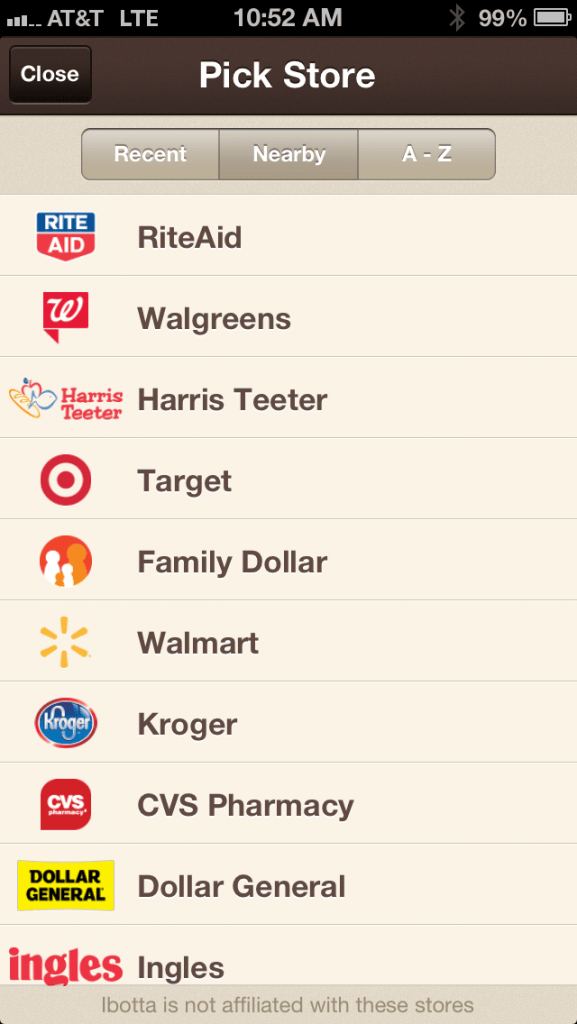This screenshot, captured on an AT&T LTE device at 10:52 AM with a 99% battery level, shows a user interface with a brown section at the top and various store listings on a tan background. The interface features a prominent Bluetooth icon and includes a brown box with white font stating "close" along with a white "pick store" button. 

The background showcases tan boxes with subtle gray shadows, with categories listed such as "recent" and "nearby" in white. Below, there's a detailed list of stores, each accompanied by its logo and name:

- **Rite Aid:** Displayed with a shield-shaped logo in blue and red.
- **Walgreens:** Featuring a red logo with a white "W."
- **Harris Teeter:** Illustrated with red letters and graphics of a loaf of bread, a red apple, and a blue fish.
- **Target:** Marked by the iconic red Target bullseye.
- **Family Dollar:** Contains an orange circle with abstract figures in white and orange.
- **Walmart:** Showcased with the gold spark symbol.
- **Kroger:** Represented by a blue circle and white "Kroger" font with a red trim.
- **CVS Pharmacy:** Sporting a red chat bubble shape with "CVS" in white.
- **Dollar General:** Identified by a yellow background with black font.
- **Ingalls:** Written in red "Ingalls."

At the bottom of the screenshot, there is a disclaimer stating, "Ibotta is not affiliated with these stores."